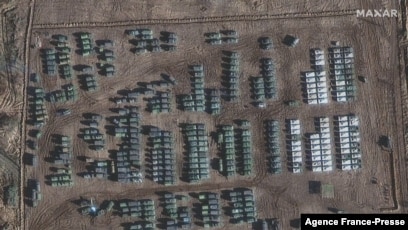This horizontally oriented, top-down satellite photograph, attributed to Maxar (top right) and Agence France-Presse (bottom right), showcases a sprawling dirt compound in a remote field. The main focus is a large, open parking lot filled with numerous vehicles, mostly aligned in straight rows, although some are scattered. The lot is a brown dirt expanse interspersed with smaller dirt roads around the perimeter. On the right side, there are white objects that could be shipping containers or buildings, adding to the intrigue of the scene. The vehicles, appearing in a greenish-gray hue, are difficult to identify due to the high vantage point, but their lined-up formation suggests organized parking. The location is ambiguous, emphasizing the isolation of this cluster of vehicles and structures in the middle of nowhere.